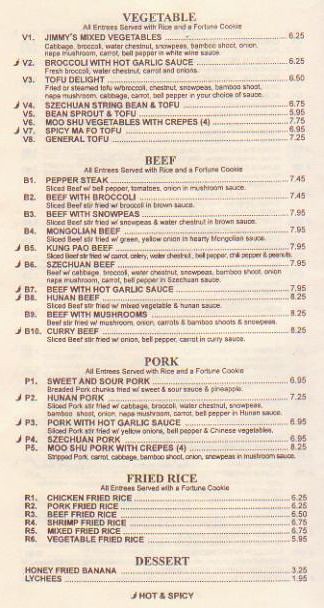This photograph captures a detailed view of a well-organized menu page from a Chinese restaurant, featuring diverse culinary offerings. The menu is divided into five distinct categories: Vegetable, Beef, Pork, Fried Rice, and Dessert. Each section presents a variety of dishes, complete with brief descriptions and corresponding indicators for hot and spicy items.

In the Vegetable section, labeled V1 to V3, the offerings include:
- V1: Jimmy's Mixed Vegetables – a medley of fresh, seasonal vegetables served with rice and accompanied by a fortune cookie.
- V2: Broccoli with Hot Garlic Sauce – a spicy dish marked with a symbol indicating its hot and spicy nature.
- V3: Tofu Delight – a savory and comforting tofu dish.

The Beef section features hearty meat dishes, listed as:
- Pepper Steak – tender beef slices cooked with bell peppers.
- Beef with Broccoli – a classic combination of beef and broccoli.
- Beef with Snow Peas – a light and flavorful dish with beef and crisp snow peas.

The Pork section, noted for its variety, includes:
- Sweet and Sour Pork – a balance of tangy and sweet flavors.
- Hunan Pork – a spicy pork dish characteristic of Hunan cuisine.
- Pork with Hot Garlic Sauce – another hot and spicy option, rich with garlic flavor.

Under the Fried Rice category, labeled R1 through R6, diners can choose from:
- R1: Chicken Fried Rice
- R2: Pork Fried Rice
- R3: Beef Fried Rice
- R4: Shrimp Fried Rice
- R5: Mixed Fried Rice – a combination of various meats.
- R6: Vegetable Fried Rice

For dessert, the menu offers:
- Honey Fried Banana – sweet, crispy banana in a light honey glaze.
- Lychees – the exotic and refreshing tropical fruit.

The prices for all dishes are attractively set under $8, making the menu not only varied but also affordable. A note at the bottom of the menu indicates that dishes marked with a specific symbol are hot and spicy, ensuring that diners are informed about the spiciness level of their choices.